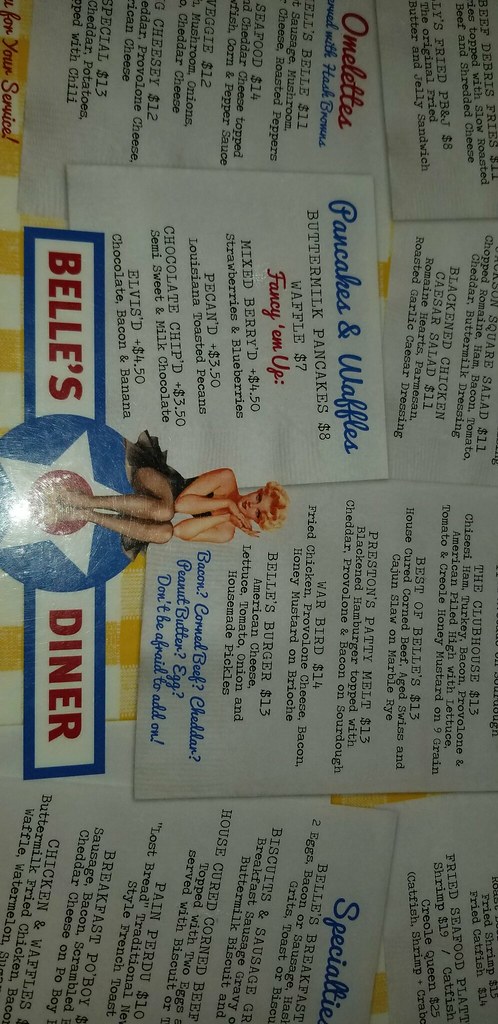This image showcases a menu from Bell's Diner, captured vertically and turned on its side. The menu is resting on a surface covered with a yellow and white checkered tablecloth. "Bell's Diner" is prominently displayed at the top of the menu, surrounded by a blue border. The text itself is white, with "Bell's" and "Diner" written in bold red letters. 

Centrally placed between "Bell's" and "Diner" is a blue circle featuring a white star with a red dot at its center. A retro pin-up style illustration of a woman, reminiscent of the 1950s, overlays the star. She is depicted wearing a strapless, short, ruffled dress and has short blonde hair.

The menu consists of multiple white pages scattered across the table, featuring blue headers and footers with red text highlights. Notable items include "Pancakes and Waffles," with buttermilk pancakes priced at $8 and waffles at $7. In red text, it states "Fancy 'em up," suggesting additional toppings like pecans or chocolate chips. Other sections visible on the menu include "Specialties" and "Entrees."